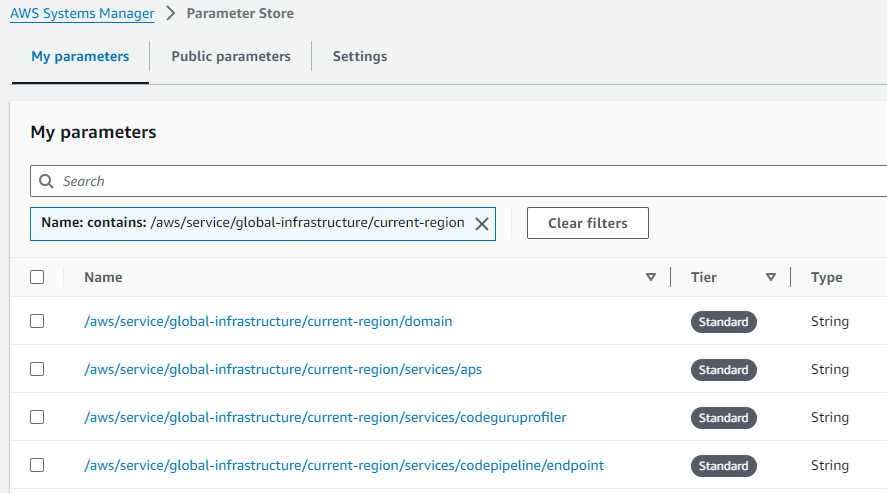The image displays a computer screen showing the AWS Systems Manager interface, specifically focused on the Parameter Store. The interface presents three main navigation options: My Parameters, Public Parameters, and Settings, with the user currently viewing the My Parameters section. At the top of this section, there's a comprehensive search bar and filtering options labeled "Name" and "Contains," already populated with terms like "AWS Service Global Infrastructure." Users have the option to clear these filters as needed.

Below the filters, the content is organized into three main columns: Name, Tier, and Type. Each entry in the Name column is highlighted in blue, indicating that they are clickable links. Next to each name, there are check boxes allowing for selection, with all entries listed as being of the 'Standard' tier and 'String' type. This layout suggests that users can manage and review different aspects of their parameters, likely relevant to various business processes. The background is generally off-white, giving the interface a clean and straightforward appearance. 

AWS, which stands for Amazon Web Services, provides a broad set of services related to business communications and infrastructure management.